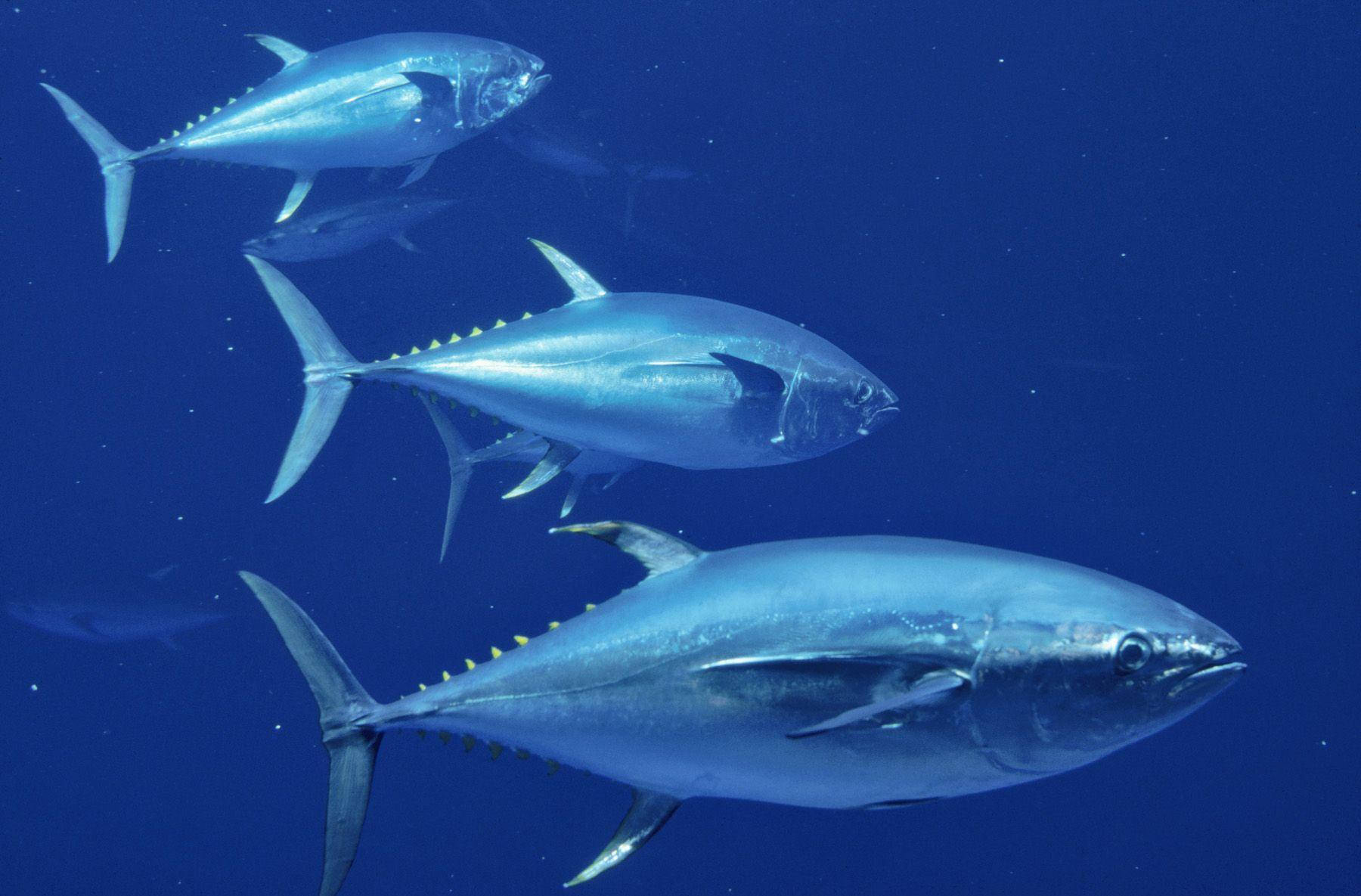The image or artwork portrays an underwater scene set against a rich, cobalt blue background, dotted with tiny white specks that suggest bubbles or particles in the water. Center stage are three sleek, streamlined fish, likely to be tuna, all oriented to the right, swimming in a somewhat staggered row. The fish have elongated, metallic-gray bodies with subtle spiny ridges along their dorsal fins, and they possess boomerang-shaped tails. A larger fish dominates the foreground, showcasing curved fins, while a slightly smaller one trails behind. The third, smallest fish swims higher up and towards the upper left corner. In the background, faint and more obscured, additional fish swim in various directions, blending into the blue water but still discernible. The overall composition highlights the orderly and serene motion of these aquatic creatures in their natural habitat.